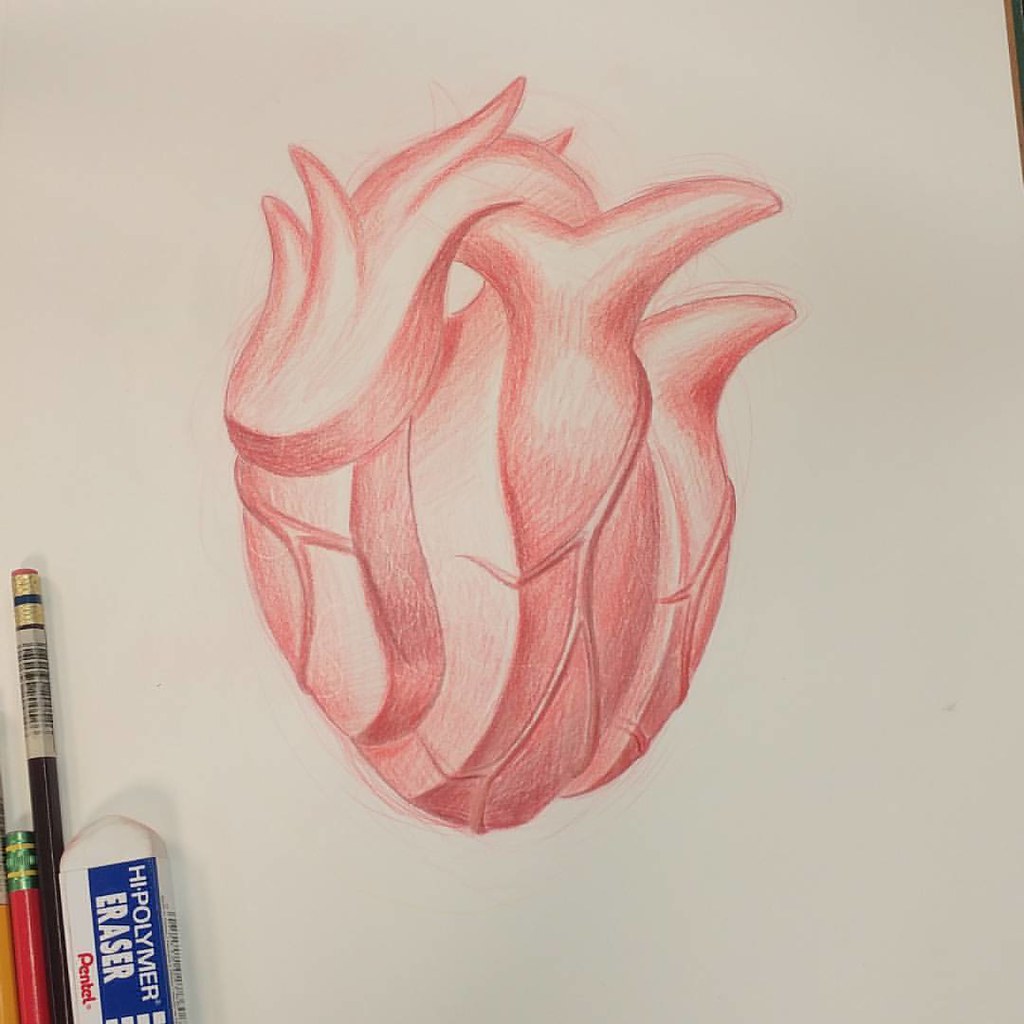The image depicts a detailed hand-drawn sketch of a human heart, created on a piece of white or light gray paper, potentially from a sketch pad. The heart is artistically rendered using a red colored pencil, with skillful shading variations distinguishing the deeper, darker outline from the lighter, more softly shaded interior. This shading technique gives the heart a dimensional, lifelike appearance. Detailed veins extend from the heart, seamlessly integrated into the red coloring.

In the lower left-hand corner of the image, the artist's drawing tools are visible, adding context to the creation process. There is a nearly used-up Pentel high polymer eraser, identifiable by its blue casing and white text, partially turned, requiring a head tilt to read. Beside it lies a red pencil worn down to the nub without an eraser, a brown pencil, and the end of a black pencil, hinting at the diverse utensils used in the artwork. The blending of varying shades of red and the meticulous detailing of the heart and its veins emphasize the artist's dedication and technique.